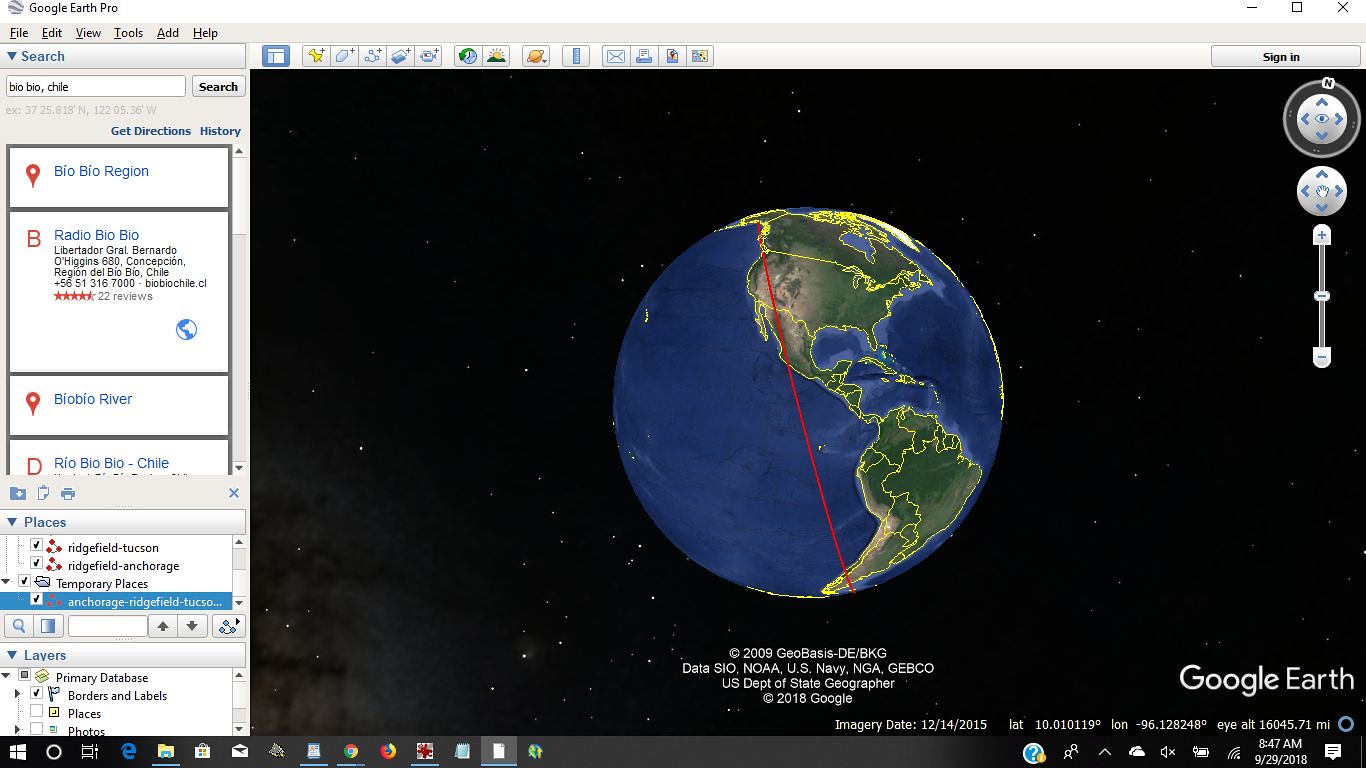This detailed screen capture showcases the browser edition of Google Earth Pro. The complete screen capture includes the top ribbon with standard Microsoft File, Edit, View, Tools, Add, and Help options. On the left side of the image, there is a vertical column of information, typical for navigation and additional options. The main focus is on the right side of the screen, featuring a 3D image of the Earth with a surrounding star field. A prominent red line runs vertically from the globe’s top to bottom, crossing the Southwest United States, Central America, and terminating near the tip of South America. The lower right corner of the image is overlaid with the "Google Earth" logo in white. The navigation buttons are clearly visible in the upper right corner, and the screen captures include all standard Windows icons and the bottom ribbon. This user appears to be navigating or exploring specific geographic data on Google Earth.